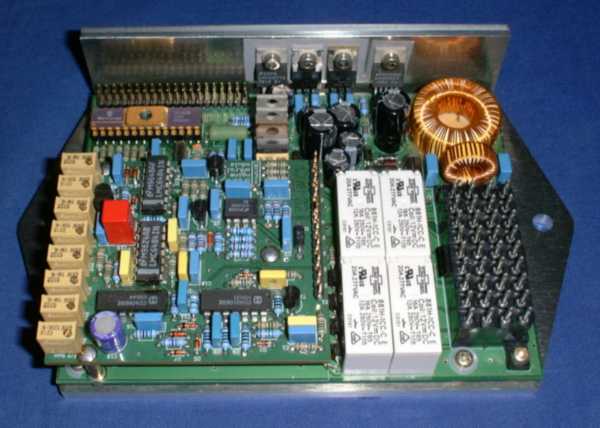The image is a detailed top-down photograph of what appears to be the inner workings of an old electronic device, possibly a computer or a fuse box. The main component is a green circuit board, partially housed in a silver metal case. The board is populated with various electronic pieces, including capacitors, coils, and fuses in multiple colors such as blue, yellow, red, tan, and white. 

On the right side of the board, there are two prominent copper coils arranged in a coil formation above four rows of what appear to be grid switches or pins. Large white rectangular boxes and smaller light brown rectangular pieces, some possibly being ports or fuses, are also visible. Other notable elements include various blue and yellow rectangles and potentially transistors. The device seems to be missing its top cover, exposing the inner components like a series of switches on a black base, further adding to the intricate layout seen in the image. 

The overall assembly, described by viewers with terms like "motherboard" and "fuse box," reflects an older type of electronic or computerized technology with a blue background surrounding it, indicating it was laid out on a blue surface for the photograph.